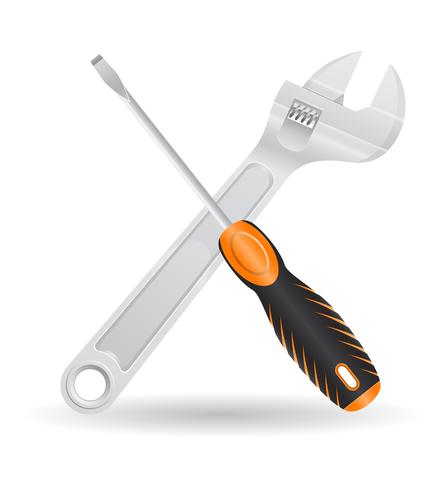The image features two tools, a silver adjustable wrench and a flathead screwdriver, arranged in a crisscross pattern against a plain white background. The wrench, devoid of any color, lies diagonally from the bottom-left to the top-right and is partially obscured by the screwdriver. The flathead screwdriver, characterized by its distinctive black and orange handle, rests atop the wrench, oriented from the top-left to the bottom-right. Underneath both tools, there is a subtle dark grey semi-circular shadow, adding depth to their presentation. The overall image, devoid of any logos, text, or additional elements, suggests a clipart style with the tools clearly being the focal point.